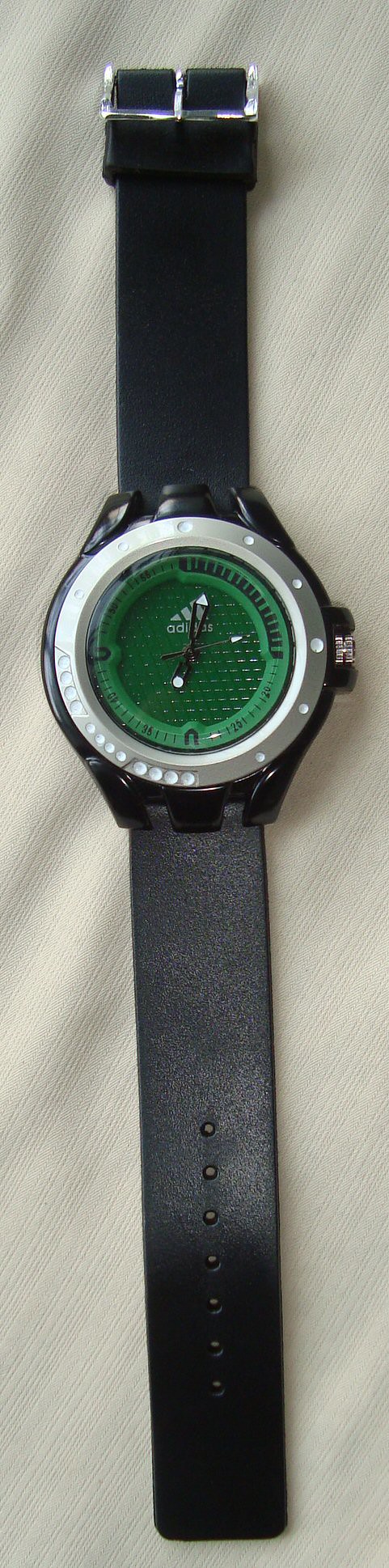This photograph features a sports watch elegantly displayed on a piece of pristine white fabric. The watch boasts a vibrant green face, encased within a sleek silver border and housed in a robust black case. The watch hands are black and appear to have a potential glow-in-the-dark feature. The watch band is a straightforward, minimalist design made from black plastic. One side of the band includes multiple perforations, while the other side is equipped with a shiny silver buckle. The overall composition highlights the watch's sporty aesthetic and functional design elements.